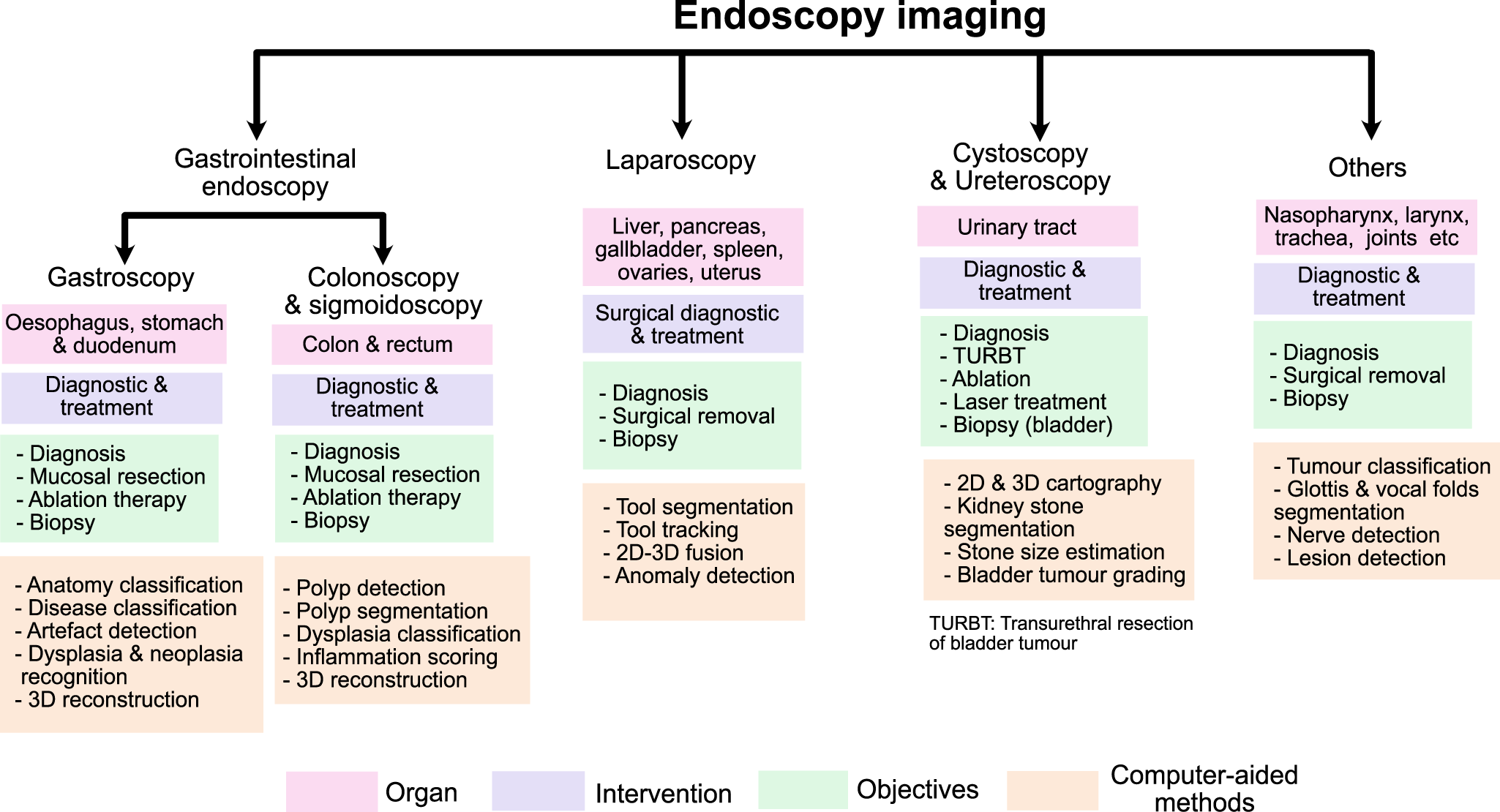The image is a detailed flowchart on a plain white background, approximately six inches wide and four inches high, designed to explain endoscopic imaging. At the top center, "Endoscopy Imaging" is written in black text. Four arrows extend downward from the text, leading to different types of endoscopy procedures: "Gastrointestinal Endoscopy," "Laparoscopy," "Cystoscopy and Ureteroscopy," and "Others."

Each primary category branches out further. For "Gastrointestinal Endoscopy," horizontal lines with arrows point downward to "Gastroscopy" and "Colonoscopy and Sigmoidoscopy." Each procedure type is associated with four rectangular boxes—colored pink, purple, green, and peach—that detail specific aspects. Pink boxes indicate organs, such as the esophagus, stomach, and duodenum. Purple boxes represent interventions, including diagnostic and treatment methods, ablation therapy, and biopsy. Green boxes define objectives like diagnosis, surgical removal, and disease classification. Peach boxes illustrate computer-aided methods like tumor classification, lesions detection, segmentation, and nerve detection.

Similarly, "Laparoscopy" deals with organs like the liver and pancreas. "Cystoscopy and Ureteroscopy" focus on the urinary tract. The "Others" category includes areas such as the nasopharynx, larynx, trachea, and joints, with corresponding diagnostic and treatment details.

A key at the bottom clarifies the color coding: pink for organs, purple for interventions, green for objectives, and peach for computer-aided methods. Each section is meticulously categorized and serves as an informative guide, ideal for educational purposes.